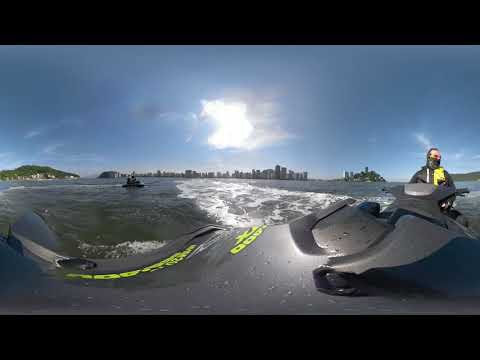The photo depicts a man on a jet ski in the ocean, prominently framed by black lines at the top and bottom of the image. The water appears dark and features white breaking waves. The man, positioned toward the right side, is wearing a black wetsuit with green and yellow accents and has a mask covering the lower half of his face. Despite a receding hairline, the top part of his face is visible. In the background, there is a distant city skyline, along with a small boat situated to the center left of the image. Additionally, there's a hilly, tree-covered island on the right, and another land mass further right. The sky above is a vibrant blue with a large, bright cloud dominating the center. At the bottom of the image is a lengthy, distorted black object with yellow lettering, featuring a large "X" followed by indecipherable characters.